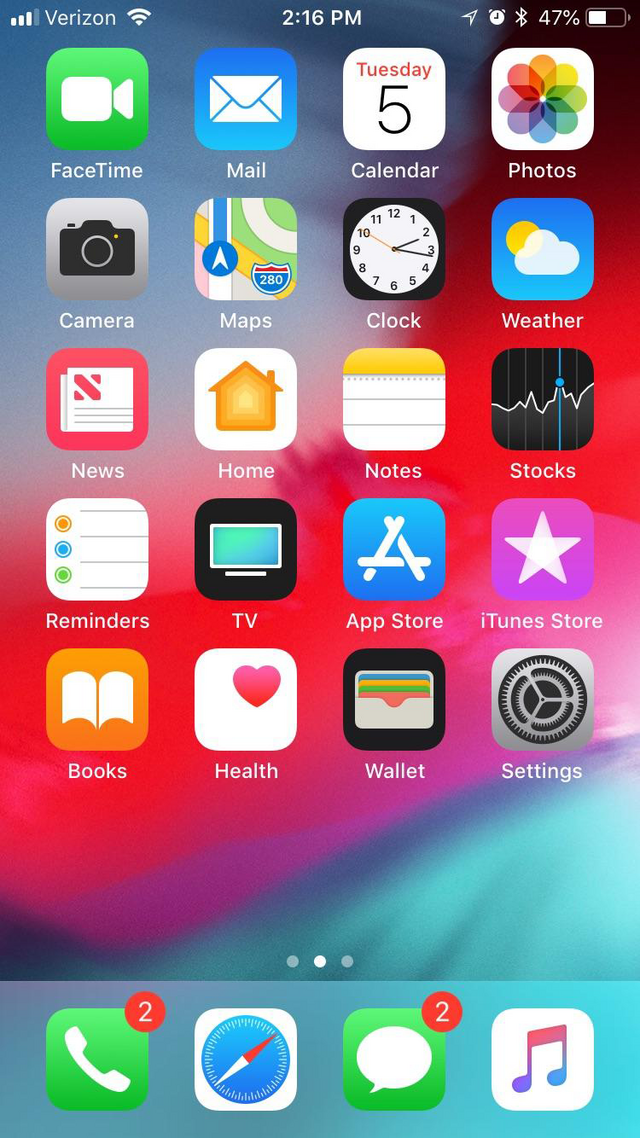A detailed screenshot of a mobile device's home screen is depicted. In the top left corner, the cell signal is displayed alongside the Verizon and Wi-Fi symbols. Centered at the top of the screen, the time reads 2:16 PM. On the top right, the status bar features location services, Bluetooth, an alarm icon, and a battery level at 47%. The background showcases a vibrant wavy color pattern, blending shades of blue, purple, pink, red, white, and bluish-gray.

The home screen layout consists of five rows of app icons (with four icons per row) and an additional row at the bottom containing four more icons. The apps displayed are:

- Top row: FaceTime, Mail, Calendar, Photos
- Second row: Camera, Maps, Clock, Weather
- Third row: News, Home, Notes, Stocks
- Fourth row: Reminders, TV, App Store, iTunes Store
- Fifth row: Books, Health, Wallet, Settings

The dock at the bottom of the screen includes the Phone, Safari, Messages, and Music apps.